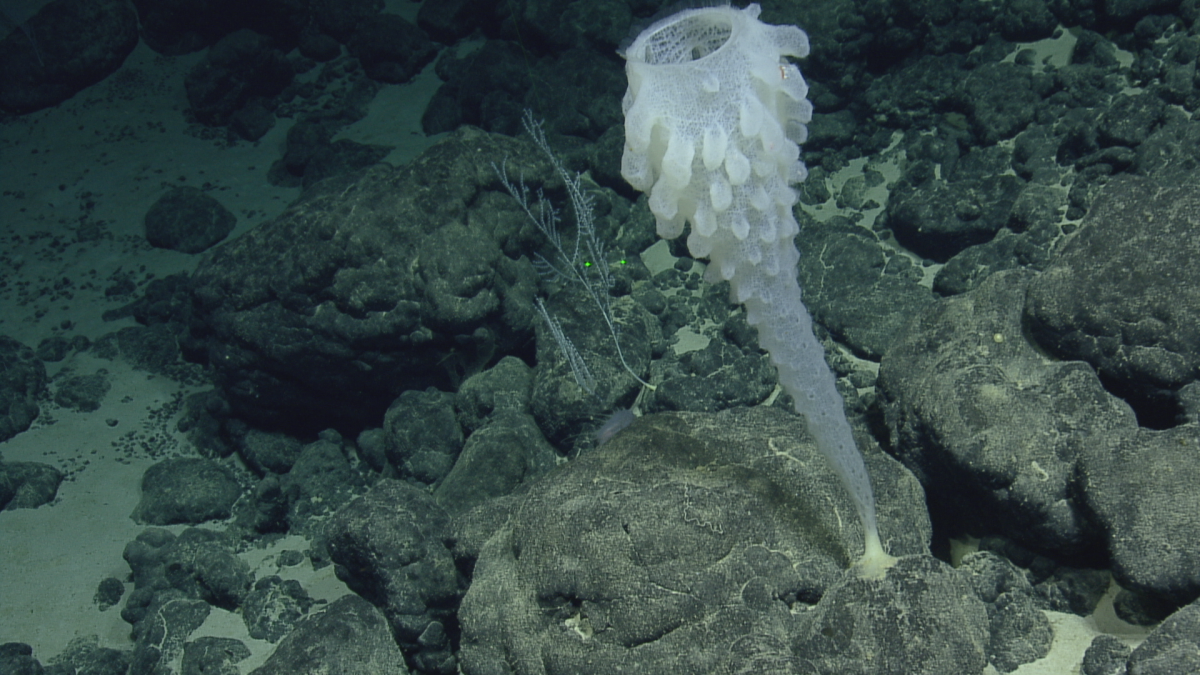The photograph captures the dark depths of the ocean floor where a muted, green hue pervades the scene. The seafloor is strewn with large, grayish rocks resembling volcanic formations, intermingled with patches of sand. Among these rocky structures, the striking feature is an enigmatic deep-sea creature attached firmly to one of the prominent foreground rocks. This creature, white and somewhat translucent, is shaped like an upside-down cone with its wider opening at the top. It appears to have tentacle-like appendages, possibly used for filtering food from the water, and is tilting slightly to the left, suggesting a gentle underwater current. In the background, faint hints of green plants add depth to the mysterious underwater landscape.